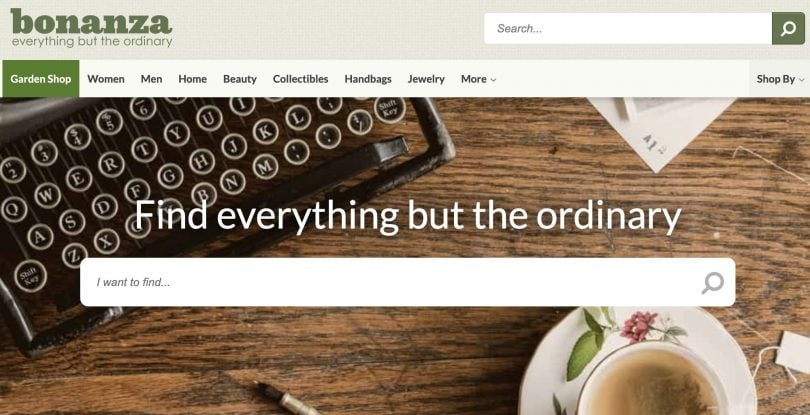The screenshot captures the homepage of Bonanza, a company highlighted by its bold, thick lowercase logo in the upper left corner, with the tagline "everything but the ordinary" in thinner, unbolded letters below it. Dominating the top section is a large rectangular white search bar accented with a magnifying glass icon. Directly beneath this, a navigational menu offers clickable links to various departments: Garden Shop, Women, Men, Home, Beauty, Collectibles, Handbags, Jewelry, and a "More" dropdown. Currently, the Garden Shop section is highlighted. The page's background features a rustic wooden desk adorned with an old typewriter—keys prominently visible—and a cup of tea resting on a saucer with a teabag peeking out. Centrally positioned within this picturesque backdrop is a large search bar with placeholder text stating, "find everything but the ordinary," followed by an invitation to enter a specific search query with "I want to find..."